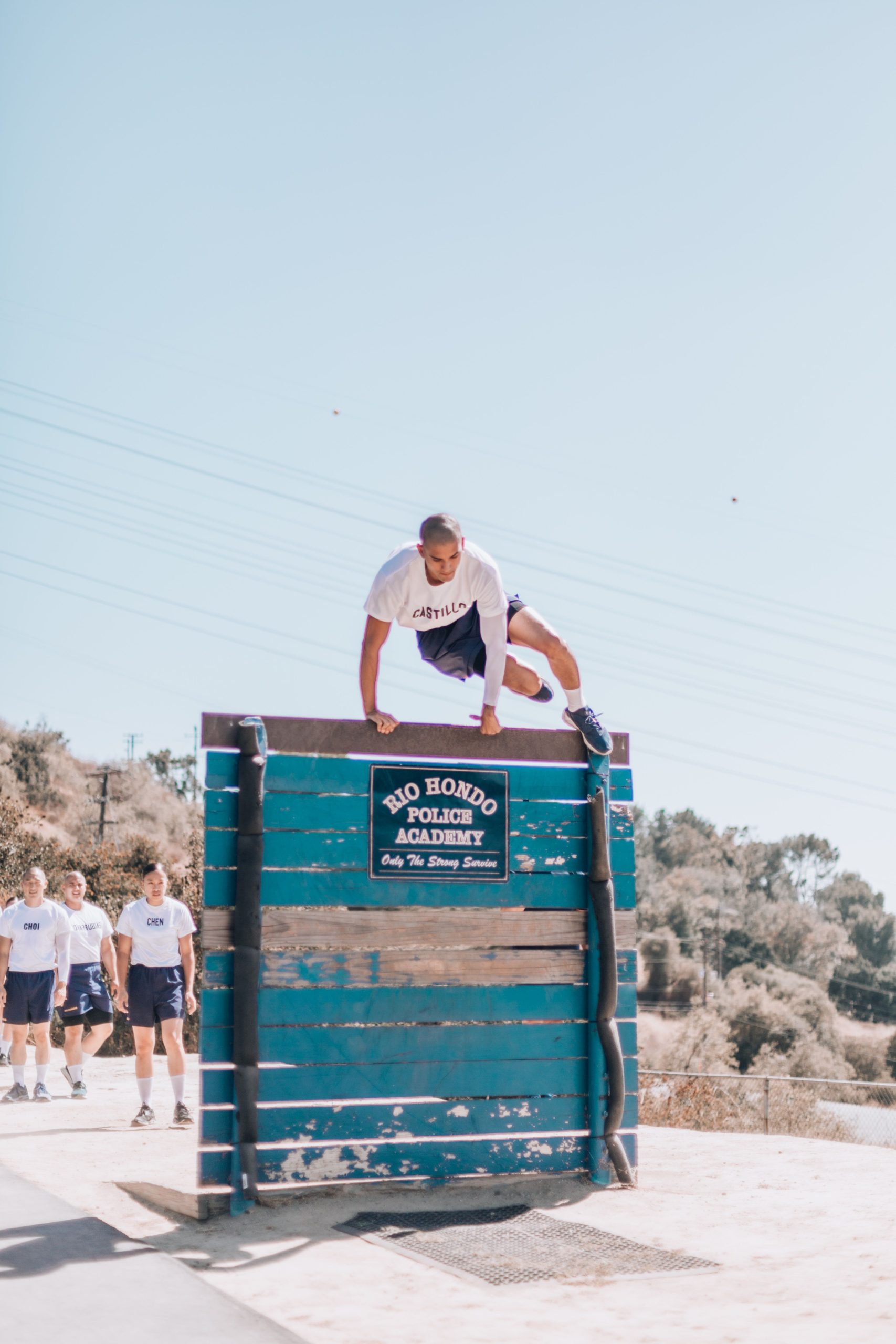The image is a color photograph in an upright rectangular orientation, capturing a training exercise at the Rio Hondo Police Academy. The central focus is a group of police recruits running up and vaulting over a tall wooden wall. The wall is constructed of multiple planks, nailed one on top of another, and is supported by vertical black bars on each side. A young man, tan-skinned and dressed in a white t-shirt, blue shorts, white socks, and blue tennis shoes, is at the top of the wall, preparing to jump over to the opposite side, which has a sign stating "Rio Hondo Police Academy" and the motto "Only the strong survive." There is a visible rubber mat or sand area for landing. Behind him, several cadets, including both men and women in identical uniforms, are lined up, ready to take their turn. The bright sunlight washes out much of the scene, indicating an intensely hot day. The backdrop features a chain-link fence enclosing the training area, with a hilly terrain covered in trees and sparse vegetation beyond.